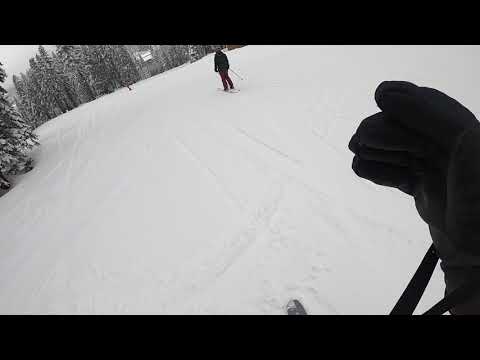The photograph captures a snowy mountain scene from the perspective of a skier. In the foreground, we see the right hand of the photographer, wearing a black glove, and the tip of his ski and ski pole barely visible in the bottom edge of the image. Directly in front of him, another skier, easily identifiable by his red pants and black coat, navigates the snow-covered terrain. The area is vast and blanketed in snow, with several trees in the background heavily coated in white. The ground appears to be an ungroomed trail with visible tracks winding down to the left. The sky, overcast and white, merges seamlessly with the snowy landscape, creating a monochromatic scene with just a hint of red from the skier's attire. The image is framed by black horizontal strips at the top and bottom, giving it a rectangular format and emphasizing the wintery, immersive atmosphere.